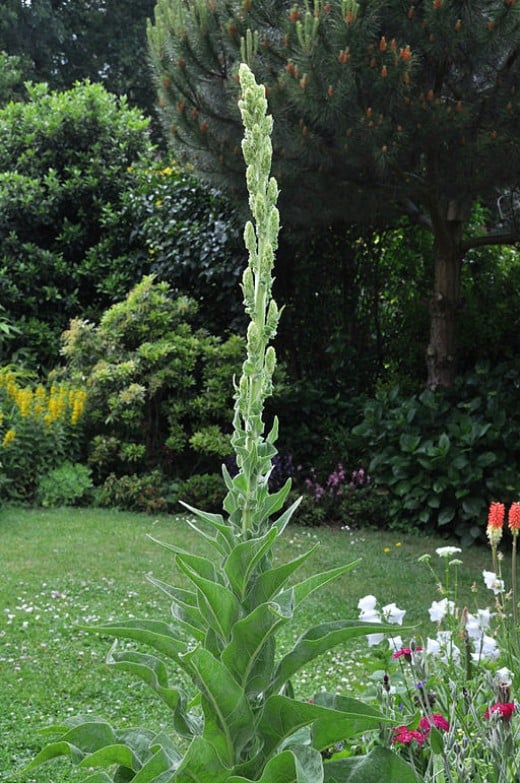The image depicts a vibrant backyard garden in full summertime bloom. The foreground features a tall, central plant standing about two to three feet high surrounded by lush green grass interspersed with little white and yellow flowers. In the bottom right corner, there is a cluster of beautiful white, pink, and red flowers adding bursts of color to the scene. Moving to the background, a stately pine tree with its brown trunk stands prominently among various shrubs and bushes, all painted in rich green hues. The setting is bright, indicative of a warm, sunny day, and overall exudes the serene and picturesque atmosphere of a well-tended garden, teeming with an assortment of colorful flowers and verdant foliage.